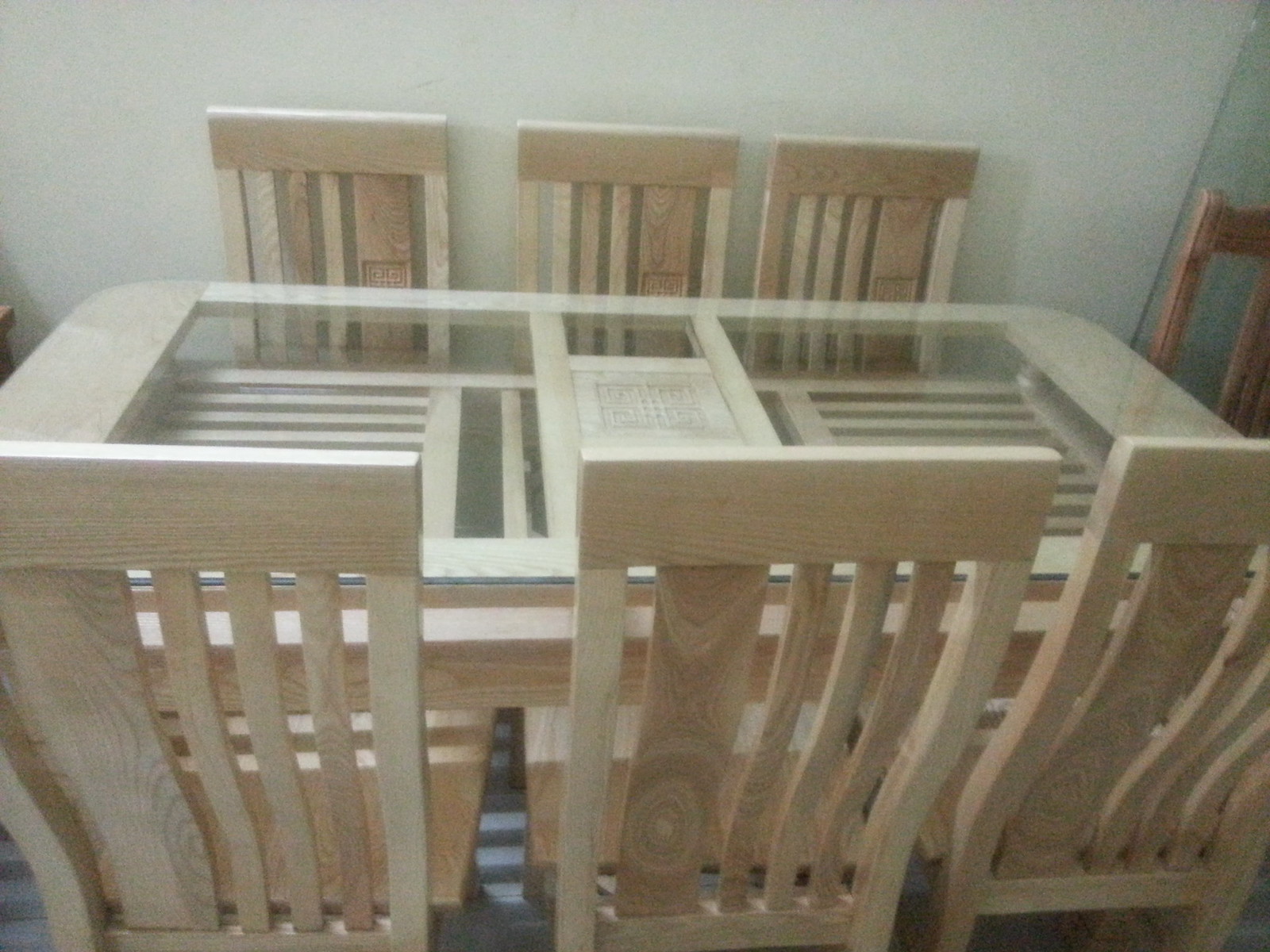This image showcases a brightly lit kitchen or dining room. Central to the scene is a wooden dining table, characterized by three glass partitions: one on the left, one in the middle, and one on the right. These glass sections are intricately designed, with small horizontal wooden slats running along them, creating a layered look. 

Surrounding the table, there are six wooden chairs, three aligned against a white wall and three more in the foreground. The chairs are in various shades of light and slightly darker brown, all appearing unfinished without any stain or paint, giving them a natural look. The top part of a seventh chair is also visible on the right edge of the image. The floor beneath the glass sections of the table is dark, enhancing the light wooden tones of the room. The tight framing of the photograph emphasizes the dining set, almost filling the entire space of the image.